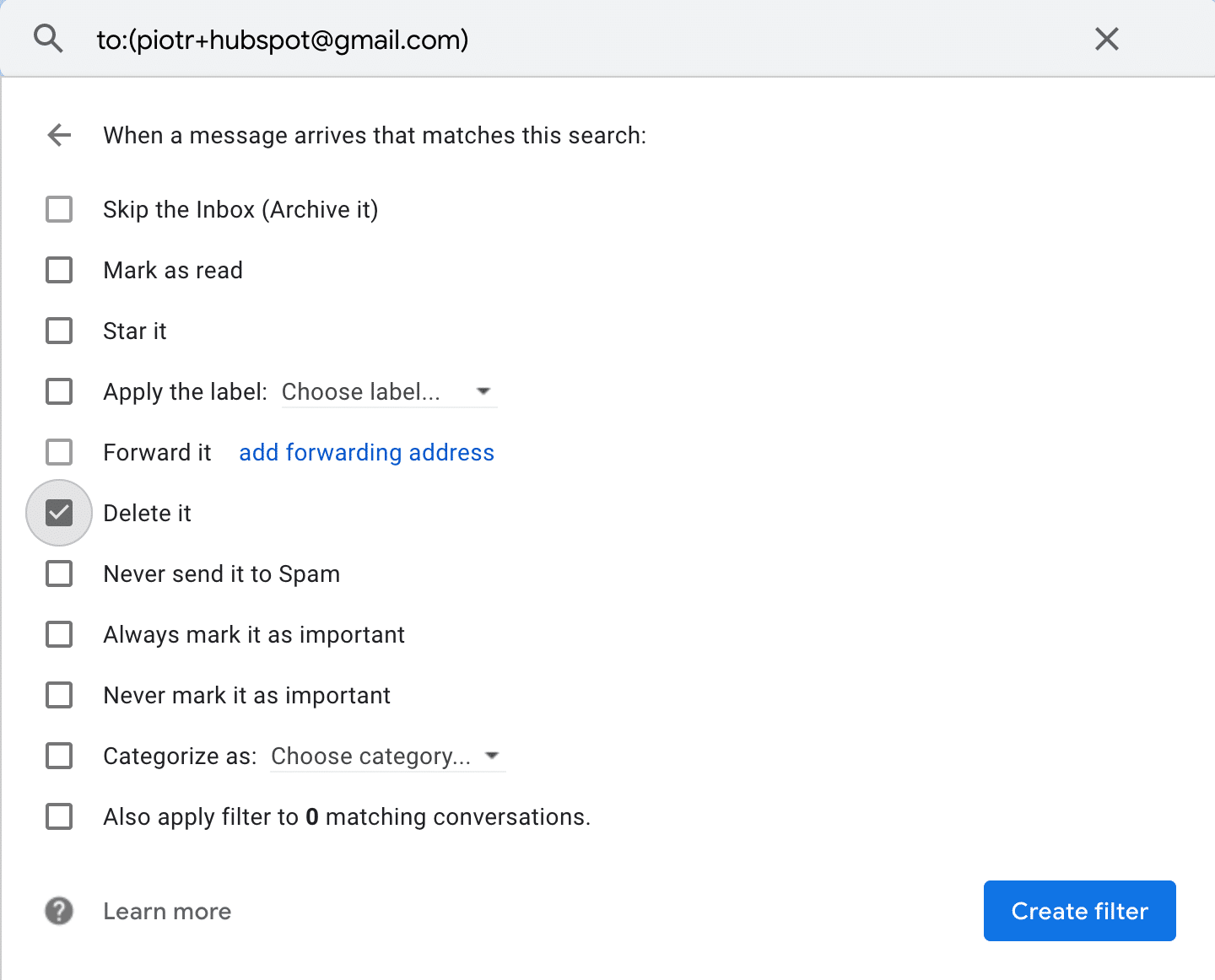The image depicts a screenshot of the 'Filters and Blocked Addresses' settings area of a Gmail account. At the top, it shows the user's email address "topileTR+hubspot@gmail.com." Below this, the section detailing how to handle arriving messages that match a specified search criteria is displayed. Several checkbox options are listed:

1. "Skip the Inbox (Archive it)"
2. "Mark as read"
3. "Star it"
4. "Apply the label: [Choose label]" (with a drop-down menu to select a label)
5. "Forward it to: [Add forwarding address]" (with a clickable blue link to add a forwarding address)
6. "Delete it" (with a checkmark already selected)
7. "Never send it to Spam"
8. "Always mark it as important"
9. "Never mark it as important"
10. "Categorize as: [Choose category]" (with a drop-down menu to select a category)
11. "Also apply filter to 0 matching conversations"

At the bottom right corner, there is a blue "Create filter" button, indicating that a new filter can be created based on the selected options.